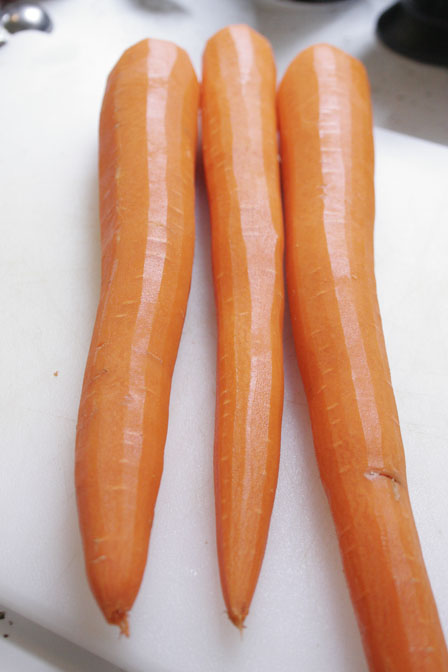The image showcases three glossy, washed, and peeled carrots of varying shapes and lengths, prominently displayed from top to bottom. The carrots, which have had their tops cut off, are vibrant orange and slightly irregular in form. They occupy the center of the frame, arrayed on a white surface that could be a chopping board or plate, against a blurred background suggestive of a kitchen. In the upper left corner, a faint, silver spherical object is visible, and the upper right corner features a blurred black circular item. The overall composition emphasizes the fresh, clean appearance of the carrots, which nearly fill the entire vertical orientation of the image.